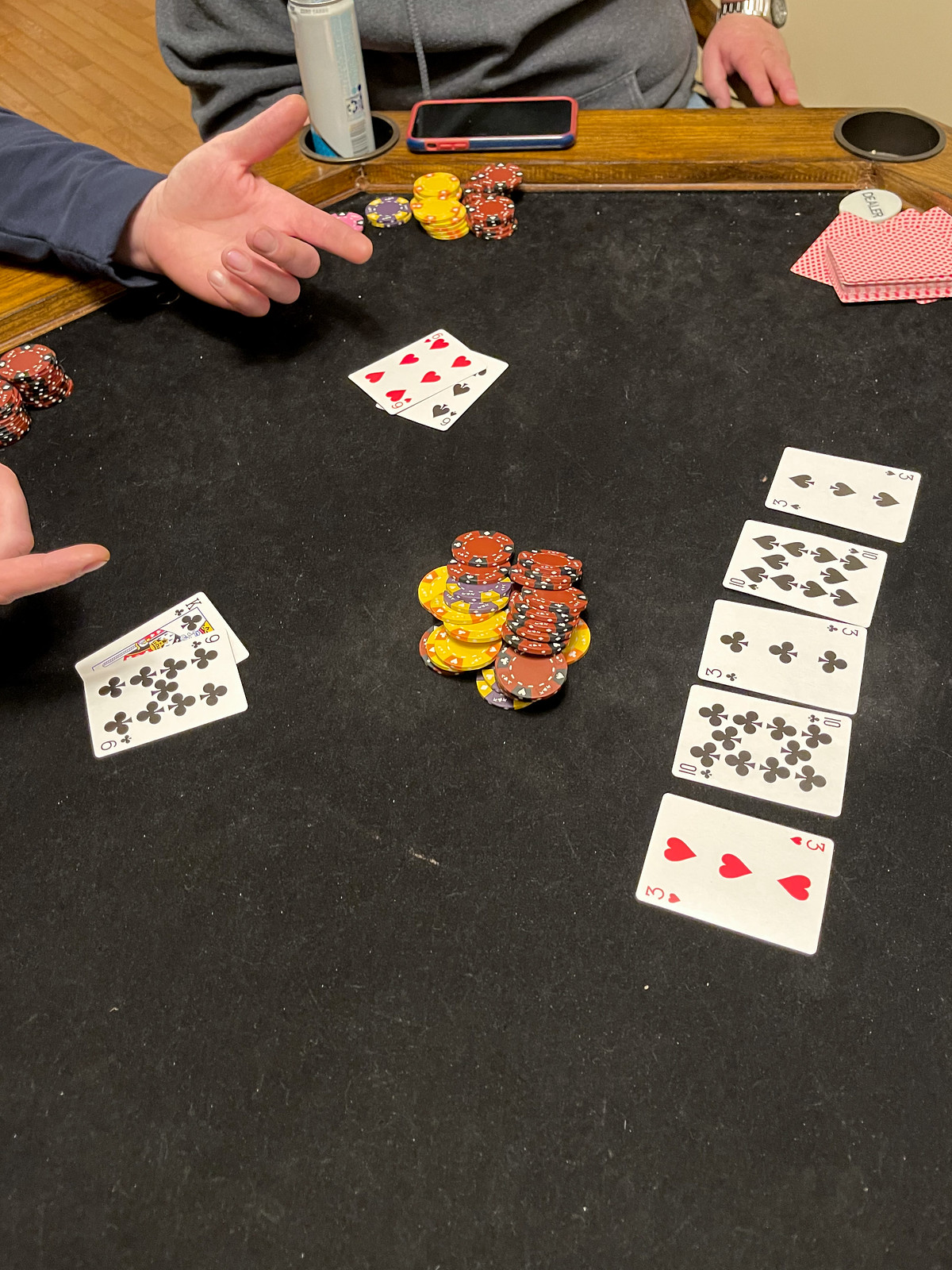A black felt-covered poker table is the central focus, laden with activity from a card game in progress. In the center, a stack of poker chips—mostly red and yellow—draws attention. The right side of the table reveals the dealer’s hand consisting of five cards: three of hearts, ten of clubs, three of clubs, ten of spades, and three of spades. 

On the left side, two player hands are visible. The top hand displays two sixes: the six of spades and six of hearts, while the bottom hand reveals a king of clubs and a nine of clubs. The upper edge of the table is made of wood, complete with cup holders for drinks, and features a cell phone resting upon it.

Scattered around the edges, more red and yellow poker chips belong to the players. In the upper right corner, the rest of the deck lies stacked face-down, their backs showing a solid red design. The scene captures the suspense and excitement of a poker game, with every detail contributing to the atmosphere.